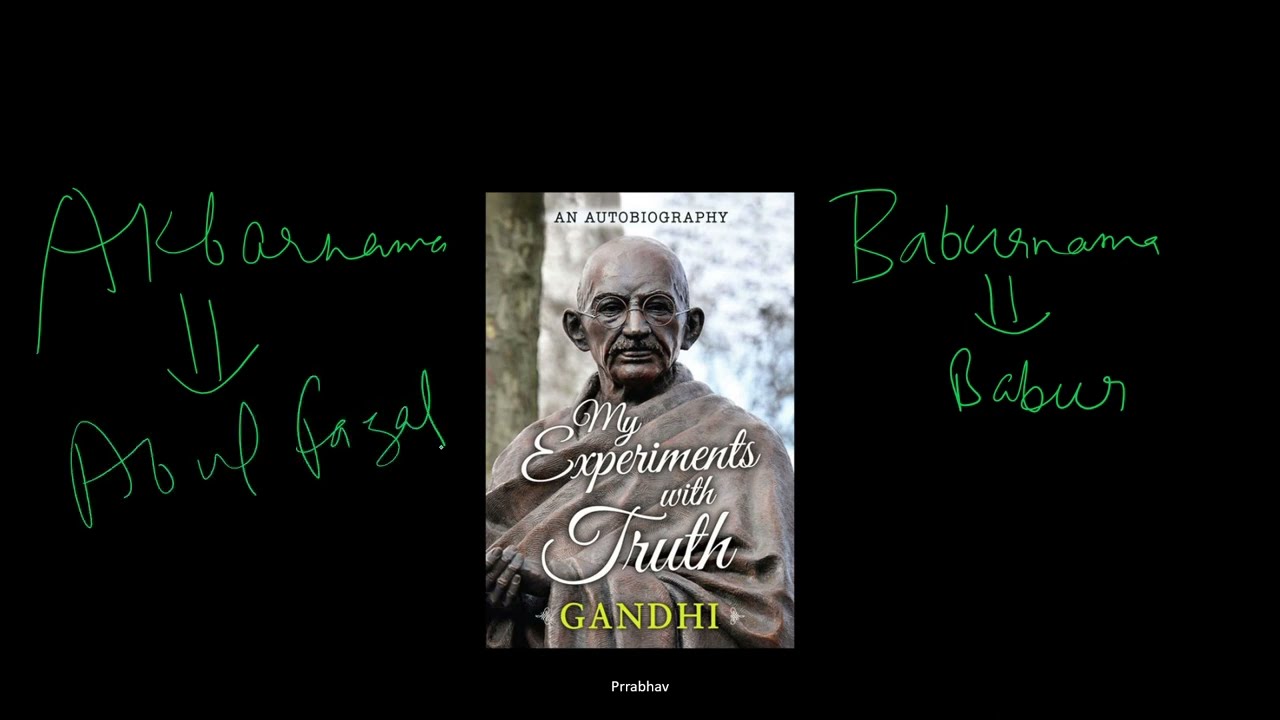The image depicts a magazine-like cover set against a large, black rectangular background. At the center, there is a picture of Mahatma Gandhi, showing him from the waist up. Gandhi, bald and dark-complected, is facing the camera with round-framed glasses, prominent ears, and a mustache. He is wearing a saggy robe and his hands are clasped together, pointing towards the lower left. 

The text on the cover is predominantly green and white. At the top, in white letters, it says "An Autobiography." Just below Gandhi's chest in white text, it reads "My Experiments with Truth." Below this, Gandhi's name is printed, in what appears to be greenish text. At the very bottom, small letters spell out "P-R-R-A-B-H-A-V."

Surrounding Gandhi's image is a background that appears to be a mix of white sky and tree trunks. Written on the black space to the left of the cover is a series of scribbles starting with "A" followed by an arrow, alongside seemingly cursive text mentioning "Aka-ba-ne-me," "Ayo-u-ba-zao," and "Abulfazal." To the right, similar green writing includes "Babu-sa-me," "Be-a-bur," and "Baburnama," both adorned with line-drawn smiley faces.